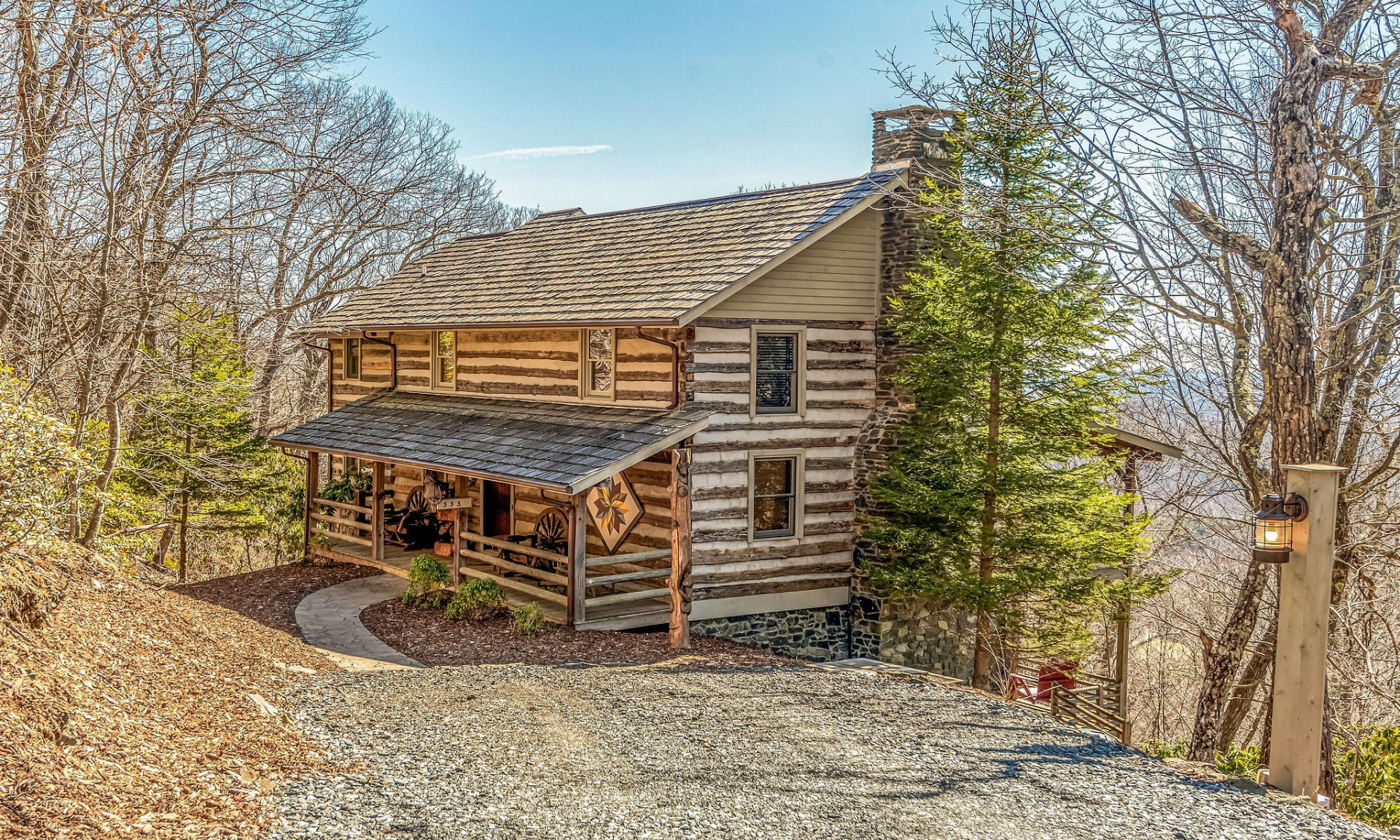This image captures a vibrant, horizontally aligned rectangular scene of a spacious, two-story log cabin nestled within a wooded mountainside. Dominated by a clear, bright blue sky, the surroundings feature predominantly leafless trees, with a few vibrant green pine trees, particularly noticeable next to the right side of the cabin. The cabin itself boasts a striking exterior of alternating light brown and dark brown horizontal wooden stripes. It’s equipped with a covered porch featuring a few rustic wagon wheels at both ends, suggesting a hint of countryside charm. The porch, partially enclosed, has someone seemingly seated beneath its shelter. 

The grounds are scattered with dead leaves and dirt, subtly highlighting a brick or stone walkway that gracefully curves to the front door. The detailed landscape comprises a driveway of gray stone and a cement path leading up to the cabin, all set amidst a multitude of natural hues like tan, beige, light and dark brown, light yellow, off-white, and multiple shades of green. To the lower right of the image, a wood post stands with a yellow-lit lamp attached, adding a warm glow to the rustic scene. This daylight photo, angled as if taken from a higher vantage point, beautifully frames the cabin and its serene, wooded environment, capturing the essence of nature and mountain retreat living.